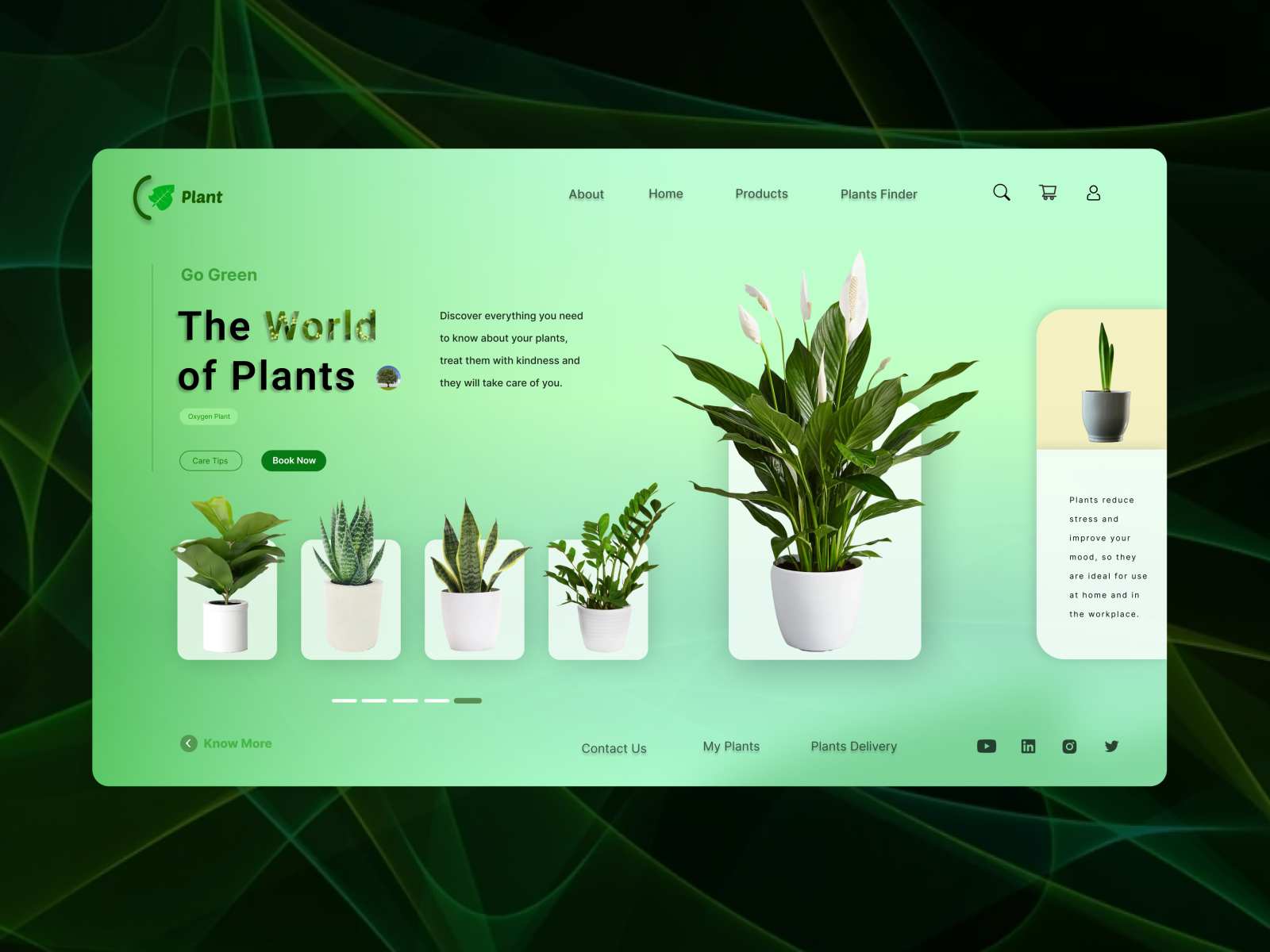This is a screenshot of a website dedicated to plants, featuring a vibrant lime green background. Prominently displayed on the web page are the words "Go Green, the World of Plants" in a welcoming font. At the top of the page, a horizontal navigation menu includes tabs labeled "About," "Home," "Products," and "Plant Finder." Beneath this menu, six images of indoor house plants, each nestled in small white ceramic pots, are neatly arranged. The accompanying text encourages the viewer with an inviting message: "Discover everything you need to know about your plants. Treat them with kindness and they will take care of you."